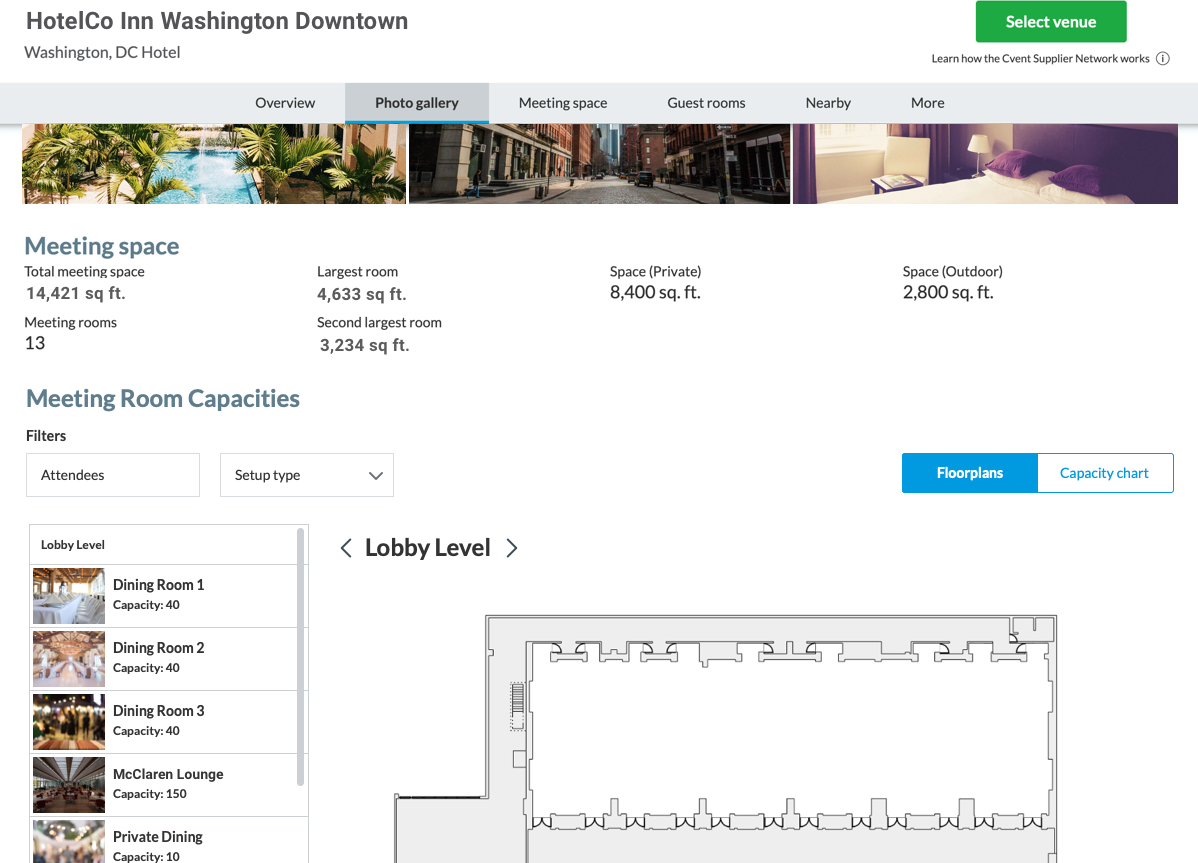This image captures the website of HotelCo, a prominent hotel located in downtown Washington, D.C. At the top right of the page, there's a green "Select a Venue" button and a link to learn about the Event Supplier Network. Scrolling further reveals several tabs including Overview, Photo Gallery, Meeting Space, Guest Rooms, Nearby, and More. The Photo Gallery tab is selected, showcasing a few images in a scrolling manner. The displayed photos include one of a pool area flanked by tropical trees, another of the bustling downtown area, and the last of a luxurious indoor room with a fancy bed. Additional details about the hotel's amenities are also visible, showing that the Total Meeting Space spans 14,421 square feet, with the Largest Room being 4,633 square feet and comprising a total of 13 Meeting Rooms. Further down, the Meeting Room Capacities are listed: Dining Room 1, 40 guests; Dining Room 2, 40 guests; Dining Room 3, 40 guests; and the McLaren Lounge, 150 guests.